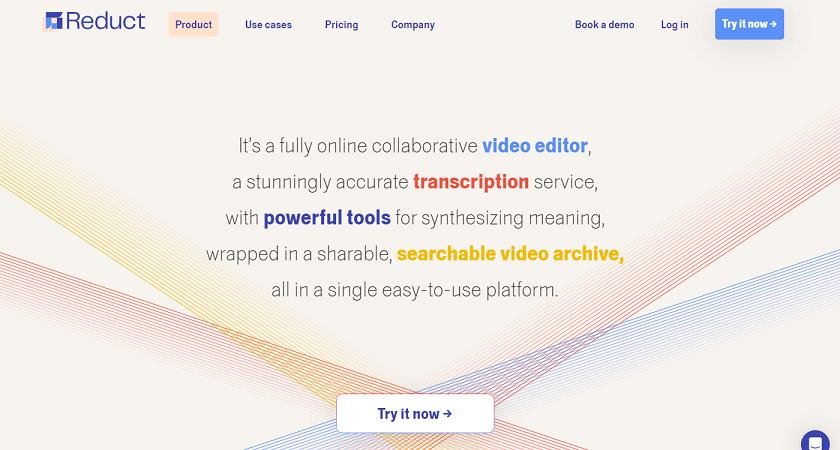The homepage screenshot of the website features a vibrant geometric background design with lines of various colors stacked at different angles. On the right, red lines ascend at a 45-degree angle, fading as they move leftward. This pattern is mirrored on the left with yellow lines. Below these, there are red lines at a shallower angle, and further down, blue lines appear at a shallower angle on the right.

Centrally located is a light beige area displaying a prominent paragraph in large text. The text describes the website as a fully online collaborative video editor and transcription service that provides powerful tools for synthesizing meaning, all within a shareable and searchable video archive on a single, user-friendly platform. Different words within the text are color-coded for emphasis: "Video editor" in light blue, "transcription" in red, "powerful tools" in dark blue, and "searchable video archive" in yellow.

Below this text, there is a white button with a multicolored outline and blue text that reads "Try it now," accompanied by a right-pointing arrow.

At the top of the page, the header continues the geometric background and features a blue logo on the left comprising two blue and two dark blue shapes on an orange square. Next to the logo, blue text reads "Reduct." To the right, blue text links include "Product," "Use Cases," "Pricing," and "Company," followed by whitespace, then "Book a Demo" and "Log In." At the far right of the header is a bright blue button with white text saying "Try it now," also accompanied by a right-pointing arrow.